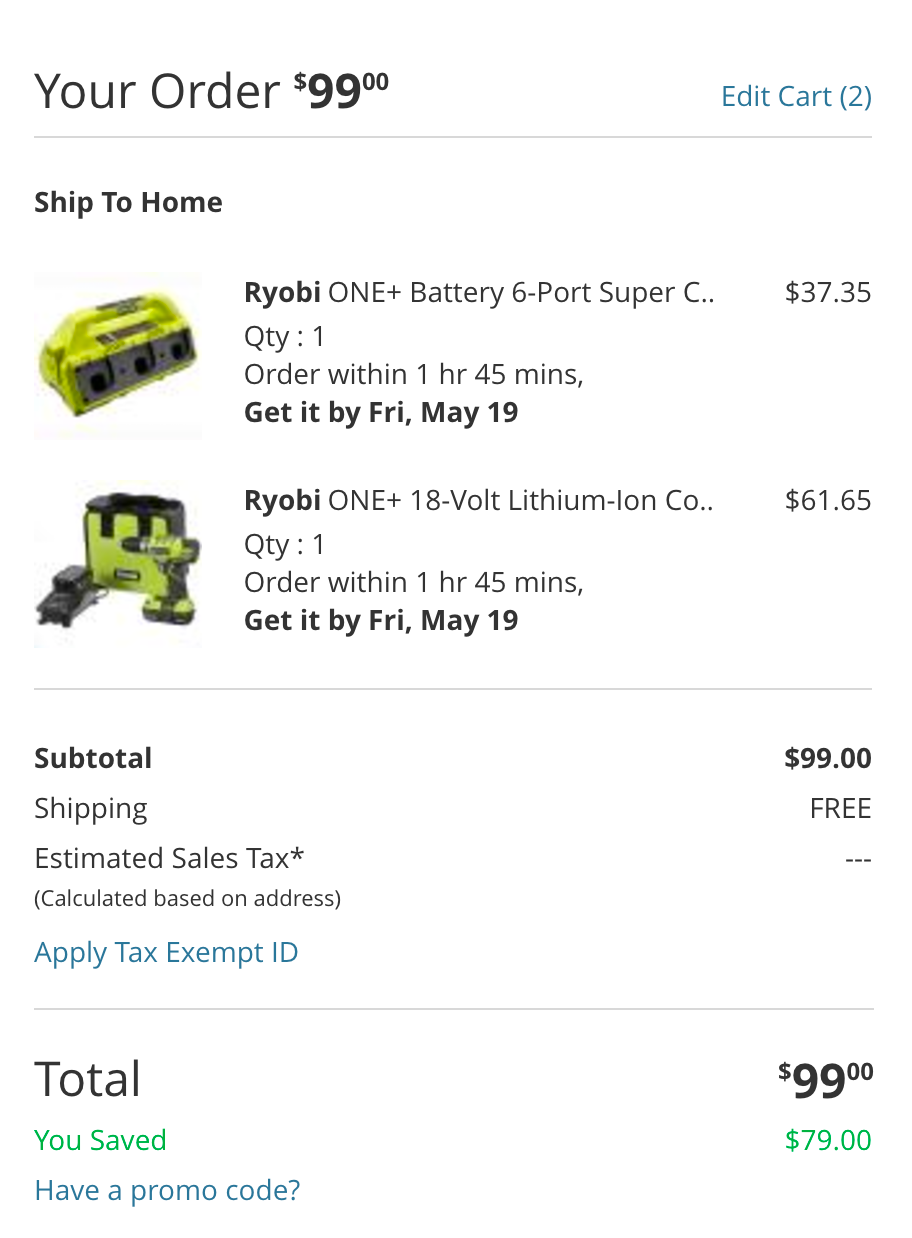This image depicts a detailed receipt page from an online order, presenting a clear summary of the items purchased and their respective costs. At the top, it indicates the total order amount as $99, accompanied by a blue hyperlink labeled "Edit Cart (2)."

The receipt states that the items will be shipped to the customer's home. The first item listed is a "Ryobi 1+ Battery 6-Port Charger," abbreviated as "Ryobi 1 Plus Battery 6 Port Super C...", with a quantity of 1. Customers are prompted to order within 1 hour and 45 minutes to ensure delivery by Friday, May 19th. The cost for this item is $37.35.

The second item is a "Ryobi 1+ 18V Lithium-Ion Cordless Drill," abbreviated as "Ryobi 1 Plus 18 Volt Lithium Ion Co...", also with a quantity of 1. The same ordering deadline and delivery date apply to this product, which costs $61.65.

On the left side of the receipt, there are pictures of both items. The image features a drill boasting a yellow and black design, accompanied by a matching case.

The summary at the bottom of the receipt details the subtotal as $99 with free shipping. It mentions that the estimated sales tax will be calculated based on the address and notes an option to apply a tax ID.